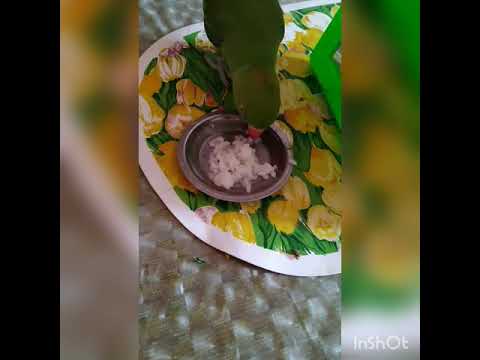In this detailed top-down image, we see a vibrant green tropical bird, possibly a parrot, pecking at some white food that resembles rice contained in a small, silver circular bowl. The bird, with its striking orange-red beak and a slight red spot on the top of its head, is positioned with its head directed towards the center of the image and its tail towards the upper part. The scene is set on a mattress with white edges, adorned with a pattern of many yellow flowers and green leaves. The mattress itself is placed on a sparkling silver surface, which could be a glass table, adding a dazzling backdrop to the vivid colors of the bird and the floral patterns beneath it.